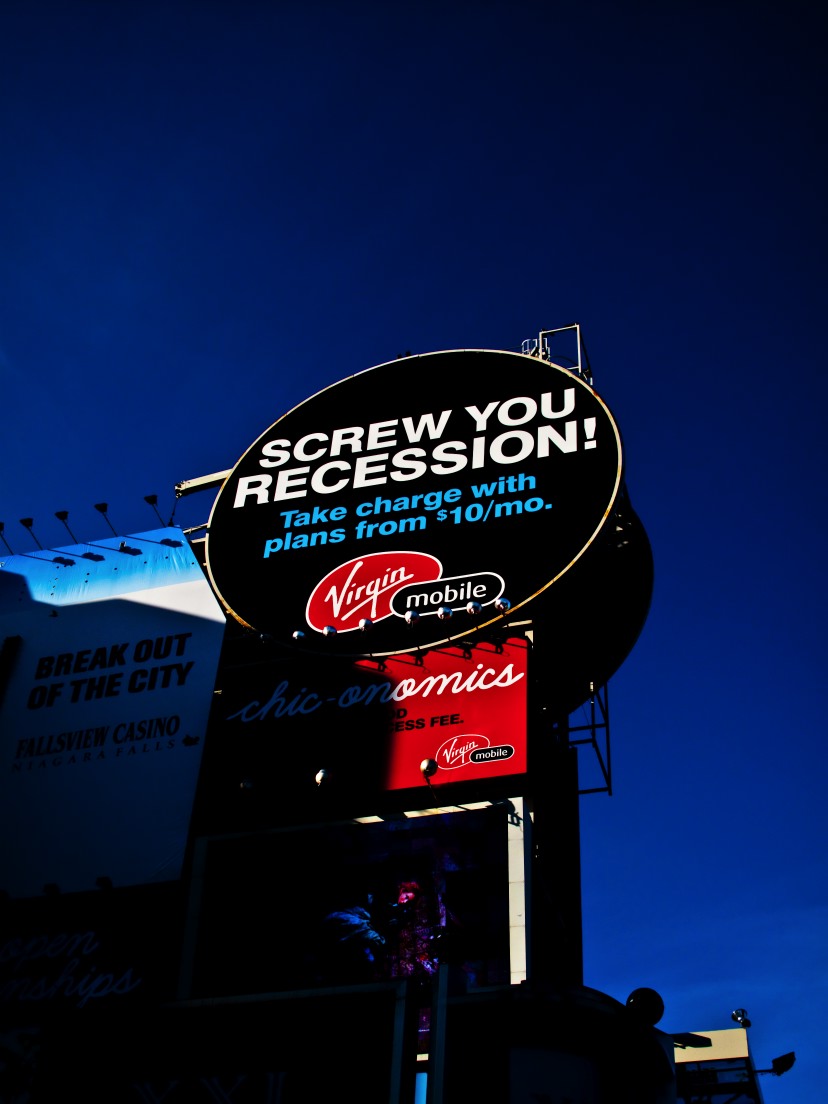This daytime photograph prominently features several segments of a Virgin Mobile billboard. The central feature is a striking black circle with white text that reads "Screw You Recession." Below this, a message in blue font states "Take Charge with Plans from $10 a Month." Further down, on a red background with white text, the iconic "Virgin" wordmark is displayed. Adjacent to this piece, a separate section on a black background shows the word "Mobile" in white font. Underneath the black circle, there's a red square with some additional white text and the Virgin Mobile logo again. Below these billboard fragments, a digital display screen is faintly visible, depicting a red and a blue figure, but its details are not entirely clear. To the side of the Virgin Mobile advertisement, another billboard is partially visible, featuring a blue top section, a white background, and some black text, likely representing a different company's ad. The image captures a bustling urban setting characterized by its layered advertising elements.